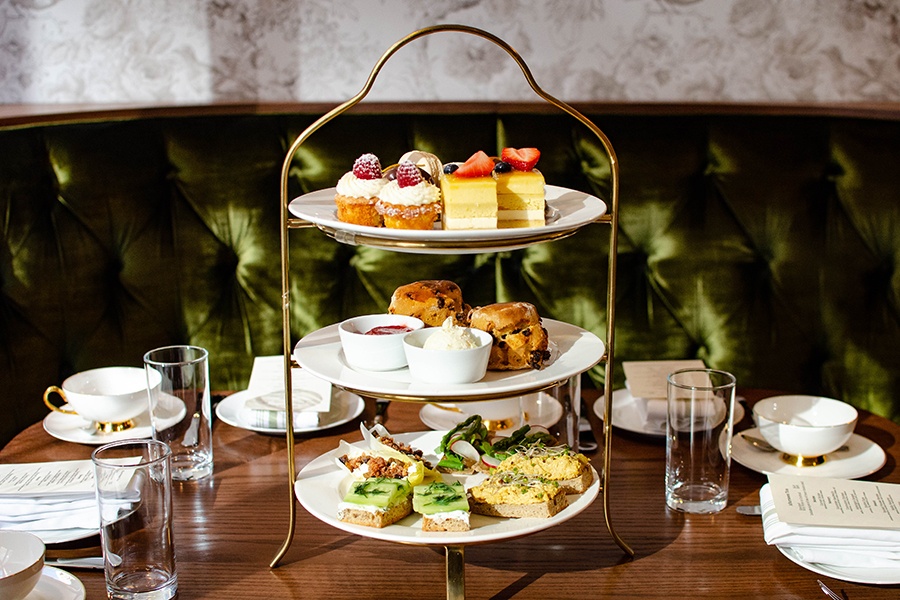This image captures a beautiful three-tiered gold stand set up for a high tea, prominently placed on a round wooden table. The stand features three circular white plates, each loaded with an assortment of delectable treats. Starting from the top plate, you can see cupcakes and layered cakes topped with fresh strawberries and other fruits. The middle plate showcases scones accompanied by small bowls of raspberry jam and whipped butter. The bottom plate hosts a variety of elegant finger sandwiches, including egg salad with cucumbers, and garnished with dill and radishes, along with some toast. The table setting includes teacups on saucers, drinking glasses, and additional plates, indicating the table is prepared for several guests. The overall scene exudes a charming and intimate atmosphere, perfect for a high tea gathering. The background is likely a wall, with no text or words present, and the overall color palette includes whites, yellows, reds, greens, browns, tans, and blacks. The image is taken indoors, although it's unclear whether it's daytime or nighttime.